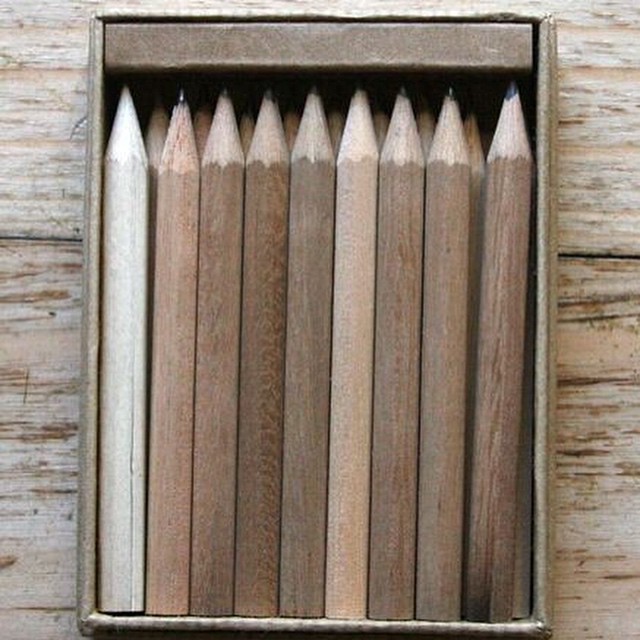The image shows a close-up of an old, brown cardboard box resembling a matchbox, containing ten short, sharpened pencils. The box rests on a rustic, worn-down wooden surface with visible scratches and splits. Each pencil exhibits slight variations in color, primarily in natural wood shades. Notably, the pencil on the far left is white or gray, and the sixth pencil from the left is lighter in color compared to the others. The pencils appear handmade or minimally processed, with one end sharpened and no erasers. Despite their worn appearance, they are barely used and fit perfectly in the box, which also features an additional rectangle piece at the top to secure the pencils in place. One of the pencils is slightly askew, hinting at a handcrafted or artisanal quality.